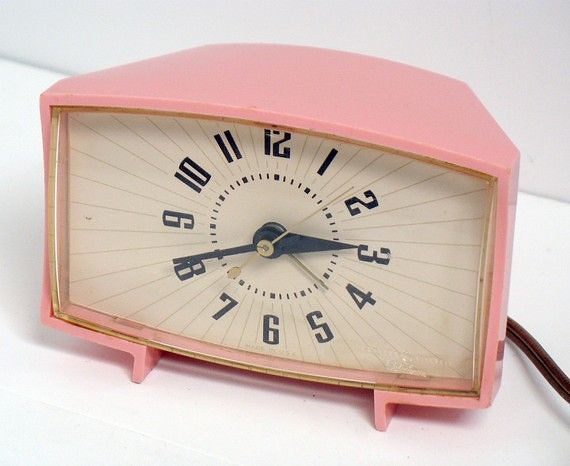The photograph features a vintage clock from the 1950s or 1960s, prominently displayed on a white stone surface. The clock, crafted from pale pink plastic, has a charmingly nostalgic appearance reminiscent of an old-fashioned television set, complete with small legs at the bottom for support. The clock face is rectangular and exhibits a classic design with numerous lines radiating from its center. The time displayed is 3:41, with the hour and minute hands in black and a gold second hand precisely ticking away. Black numbers clearly mark the hours, and an additional circular dial beneath the numbers seems to indicate half-second intervals. A brown cord extends from the back of the clock, suggesting it is electric. The background features a plain white wall, emphasizing the clock's vintage aesthetic against the minimalist setting.